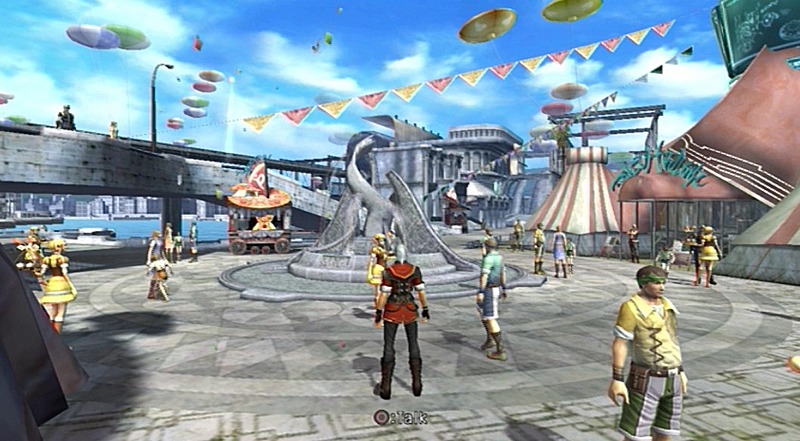In this vibrant screenshot from a video game, a lively festival scene unfolds under a clear blue sky dotted with fluffy white clouds. The ground is paved with gray tiles featuring an intricate geometric pattern, incorporating diamonds and circles adorned with pinwheel shapes. Dominating the center of the scene is an ornate gray statue of a dragon, exuding a sense of mythical grandeur. To the right, a circus tent in bright red and white hues stands out, adorned with red and yellow banners and festooned with triangular pennants, evoking a cheerful and festive atmosphere.

In the middle of the screen, a character dressed in a striking outfit catches the eye. Clad in black pants and shoes, the character's distinctive top features a bold red and black design, accented with what appears to be silver elements, adding a hint of elegance. Below the character, an icon with a red circle and the word "Talk" indicates an interactive element, inviting players to engage with the surroundings and characters.